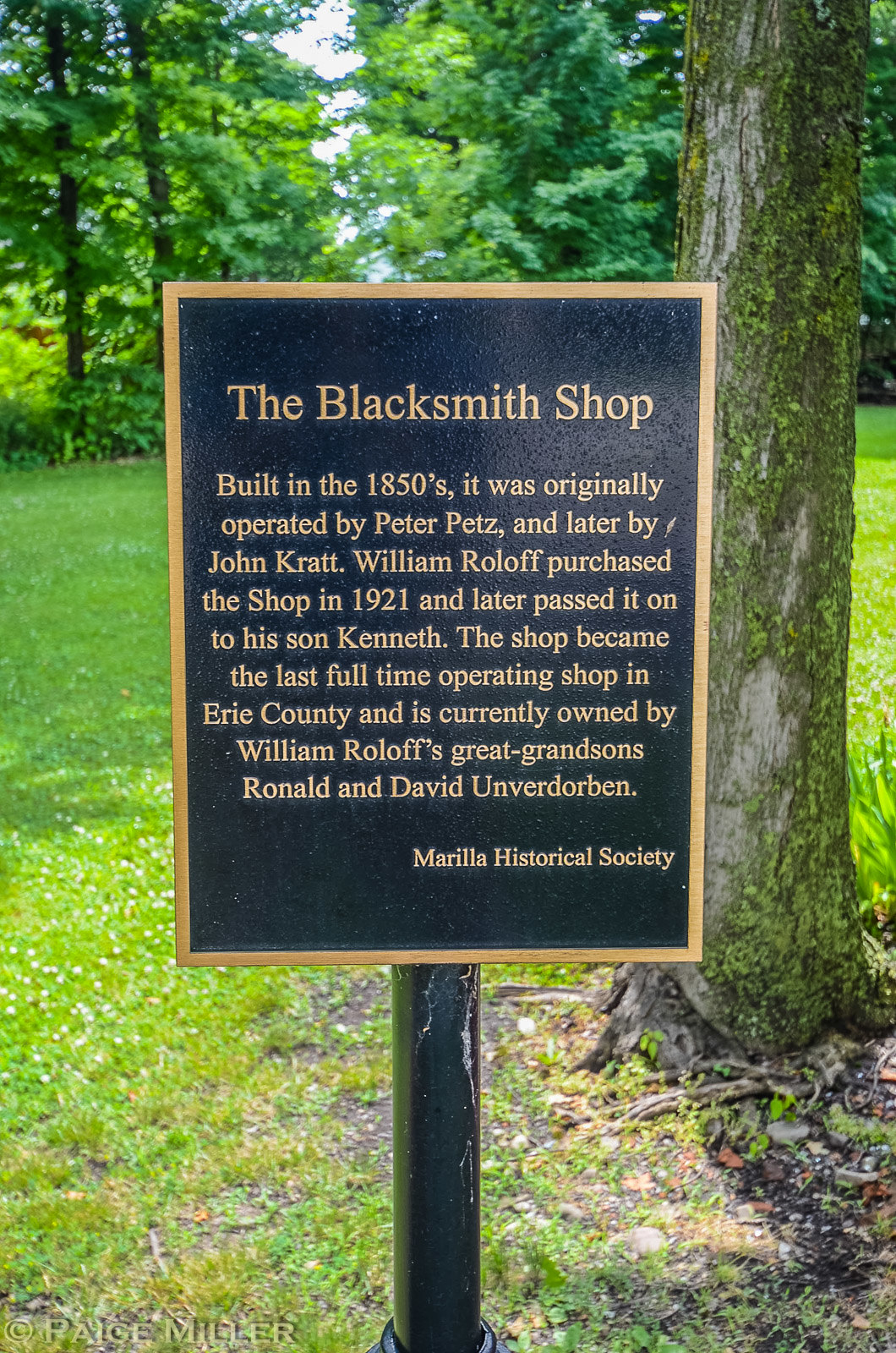The image captures an outdoor scene with a grassy area in the foreground and several trees both close and in the background. Prominently, there is a black metal plaque mounted on a black post, which is bordered in gold and bears gold text. The plaque is positioned beside a tree trunk adorned with moss and small weeds. The title on the plaque reads "The Blacksmith's Shop," followed by detailed history: "Built in the 1850s, it was originally operated by Peter Petz and later by John Craft. William Roloff purchased the shop in 1921 and later passed it on to his son, Kenneth. The shop became the last full-time operating shop in Erie County and is currently owned by William Roloff's great-grandsons, Roland and David Unverdorben." At the bottom of the plaque, it states "Marilla Historical Society." In the backdrop, the bright sky filters through the leaves of tall surrounding trees, enhancing the lush, verdant setting. The plaque additionally features a watermark with the photographer’s name, Paige Miller, at the lower left corner.